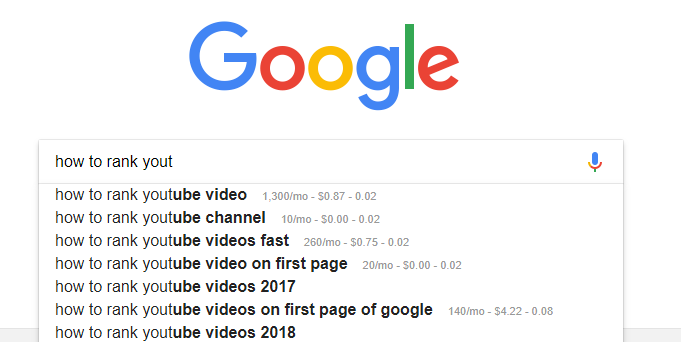The image showcases a graph from Google, featuring the iconic Google logo at the top center. The logo is displayed in the signature Google colors: the capital 'G' in blue, the first 'o' in red, the second 'o' in yellow, the second 'g' in blue, the 'l' in green, and the 'e' in red. Below the logo is a search bar with a drop-down menu displaying several autocomplete suggestions related to ranking YouTube videos. The suggestions listed are: "how to rank YouTube video," "how to rank YouTube channel," "how to rank YouTube videos fast," "how to rank YouTube videos on first page," "how to rank YouTube videos 2017," "how to rank YouTube videos on first page of Google," and "how to rank YouTube videos 2018." Next to each suggestion, except for "how to rank YouTube videos 2017" and "how to rank YouTube videos 2018," there are monthly search volume numbers and associated costs, presented in descending order. A microphone icon is visible on the right side of the search bar, indicating the option for voice search.